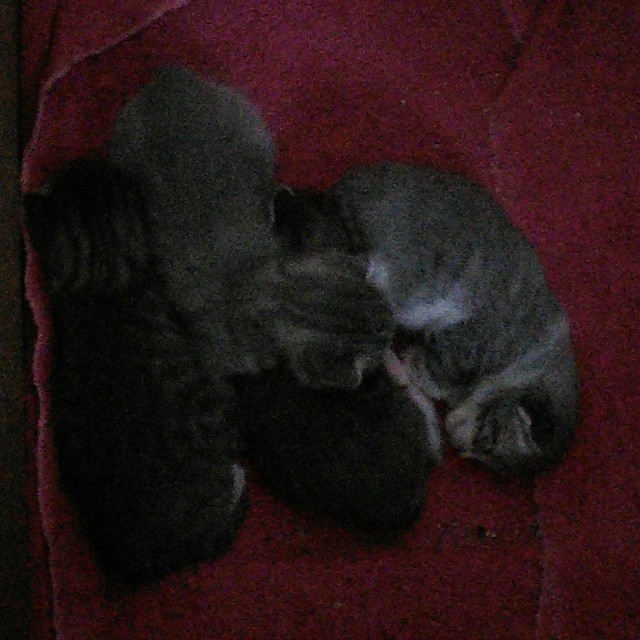This heartwarming photo captures four small kittens, peacefully sleeping on a rich, dark red towel, which seems to have a bit of black in it. The image is grainy and blurred, with a dimly lit room adding to the cozy atmosphere. Two of the kittens have dark gray or almost black fur, while the other two are primarily gray with black stripes on their heads. The dark kittens are positioned with their heads towards the top of the photo. Nestled between them, one gray kitten rests its head on the neck of the second dark kitten, creating a snug and adorable cluster. The fourth gray kitten, distinguished by a bit of white on its foot, lies with its head pointed towards the bottom of the frame. Additionally, some kittens show patches of white on their stomachs or around their feet. Altogether, the affectionate arrangement and the soft details of their fur make this an incredibly endearing scene.